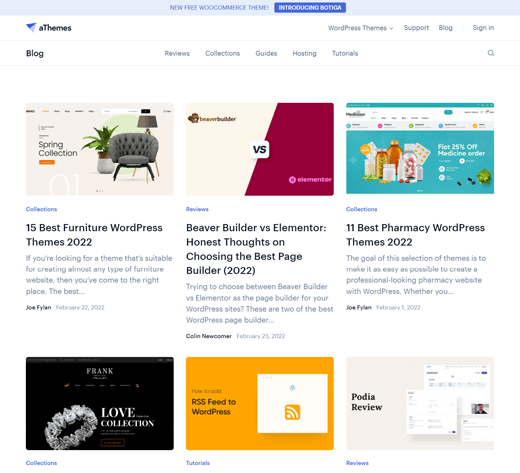The image depicts a detailed screenshot of the A-Themes website, identifiable by its distinctive logo featuring a paper airplane with one wing in dark blue and the other in light blue. At the top, a prominent banner announces a "New free WooCommerce theme: Introducing Bottega." Below the banner, the main navigation menu displays links to "WordPress Themes," "Support," "Blog," and "Reviews." 

The blog section is open, revealing further subsections including "Reviews," "Collections," "Guides," "Hosting," and "Tutorials." The page displays a variety of blog entries with accompanying images and headlines. Prominent examples include "15 Best Furniture WordPress Themes, 2022," illustrated with a picture of a couch, and "11 Best Pharmacy WordPress Themes," featuring a photo of medications. The layout includes generous white space, enhancing readability and visual appeal.